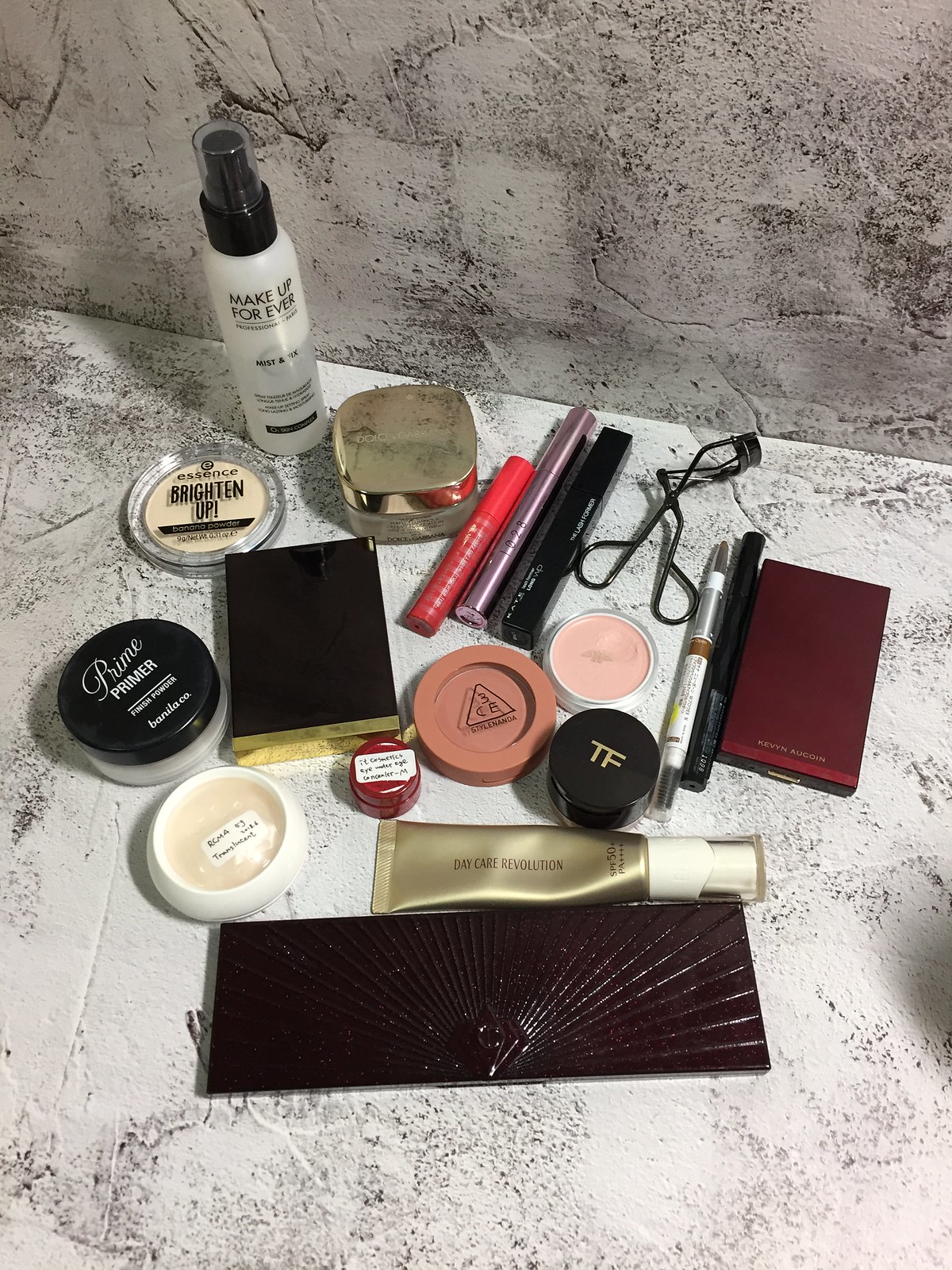A meticulously arranged collection of makeup products is displayed on a textured, predominantly white stone surface adorned with gray bubbles and cracks, set against a stone wall. The diverse array of items includes several makeup palettes and eyebrow pencils, a pencil sharpener, an eyebrow straightener, a bottle of makeup mist, a primer, and a small tube, each item positioned closely together. Notably, the circular makeup items are situated toward the rightmost edge and the center of the surface, while the square-shaped products are placed toward the back and near the central area. The pencils, on the other hand, are neatly lined up against the wall in the middle, adding a sense of order to the assortment. This composition evokes an organized yet dynamic scene, highlighting the variety and utility of the makeup tools.